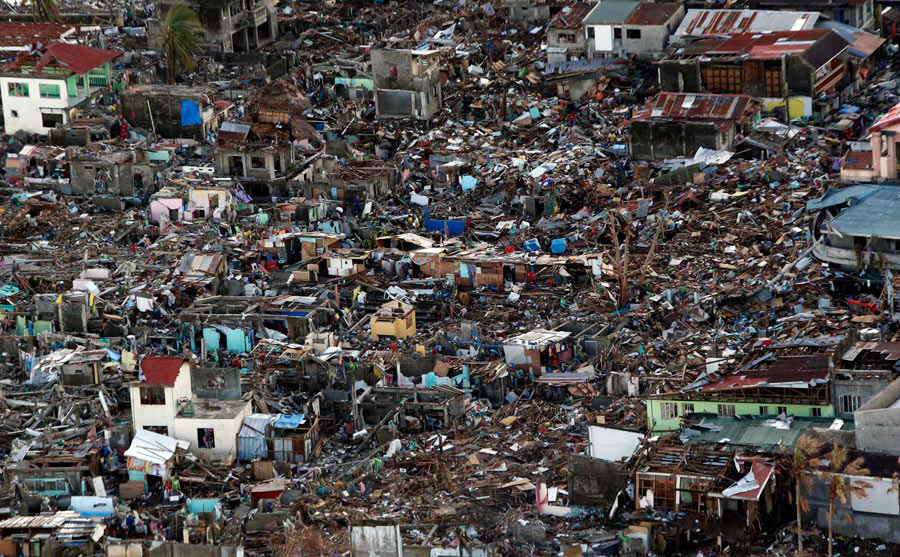The image depicts an aerial view of a hillside city slum that appears to have been severely impacted by a natural disaster, possibly a tsunami, earthquake, or hurricane. The ground is obscured by debris, with structures and homes in various states of destruction. Some homes have white or gray facades, while others include splashes of green, blue, red, and yellow, though many are in shambles. The scene is characterized by fragmented pieces, fallen debris, and wreckage scattered everywhere, suggesting the area was hit hard by the catastrophe. A few homes on the outskirts remain standing, showcasing thin, fragile structures contrasted by the decimated buildings in the center. Amidst the devastation, people can be seen sifting through the rubble, highlighting the dire situation and the extensive loss suffered in this seemingly impoverished neighborhood.